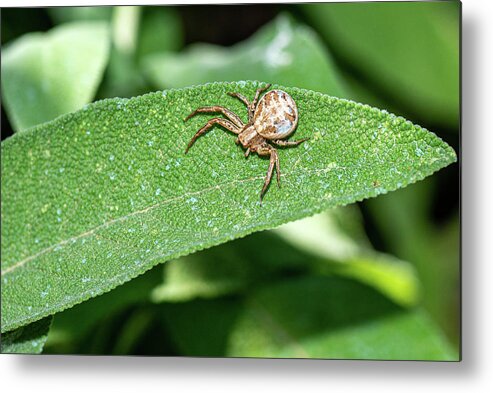This is a close-up photo showcasing a thin, elongated, sage-like green leaf with a bumpy texture and a prominent whitish vein running down the center. Resting on the leaf is a unique, cream-speckled brown spider with a bulbous abdomen adorned with possible side-to-side rounded stripes of varying shades of brown and white. The spider appears small and is resting comfortably, perhaps sunning itself. In the background, you see an out-of-focus array of green leaves, with a hint of yellow, enhancing the focus on the intricate details of the leaf and its unusual arachnid visitor. The spider's legs are splayed out, adding to its distinctive and somewhat flattened appearance.